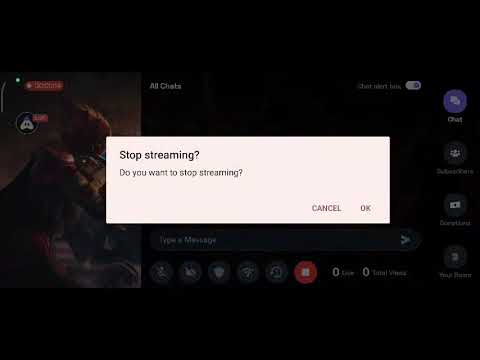The image displays a computer desktop screen dominated by a prominent white notification box at the center, which reads "Stop streaming? Do you want to stop streaming?" with "Cancel" and "Okay" options in the bottom right. The background is mostly black and features a darkened scene, including a sci-fi character with a red cloak or helmet, partially obscured. Icons and menu options scattered around the screen suggest streaming tools, such as those for Wi-Fi, chat, and audience interaction. In the top left of the background, the word "Chats" is visible, while the right side hosts a vertical list of clickable buttons labeled "Chat" with a blue tint, and a small person icon. Below the notification box, there is a red button marked with "Stop streaming" alongside related zero indicators and other small icons.